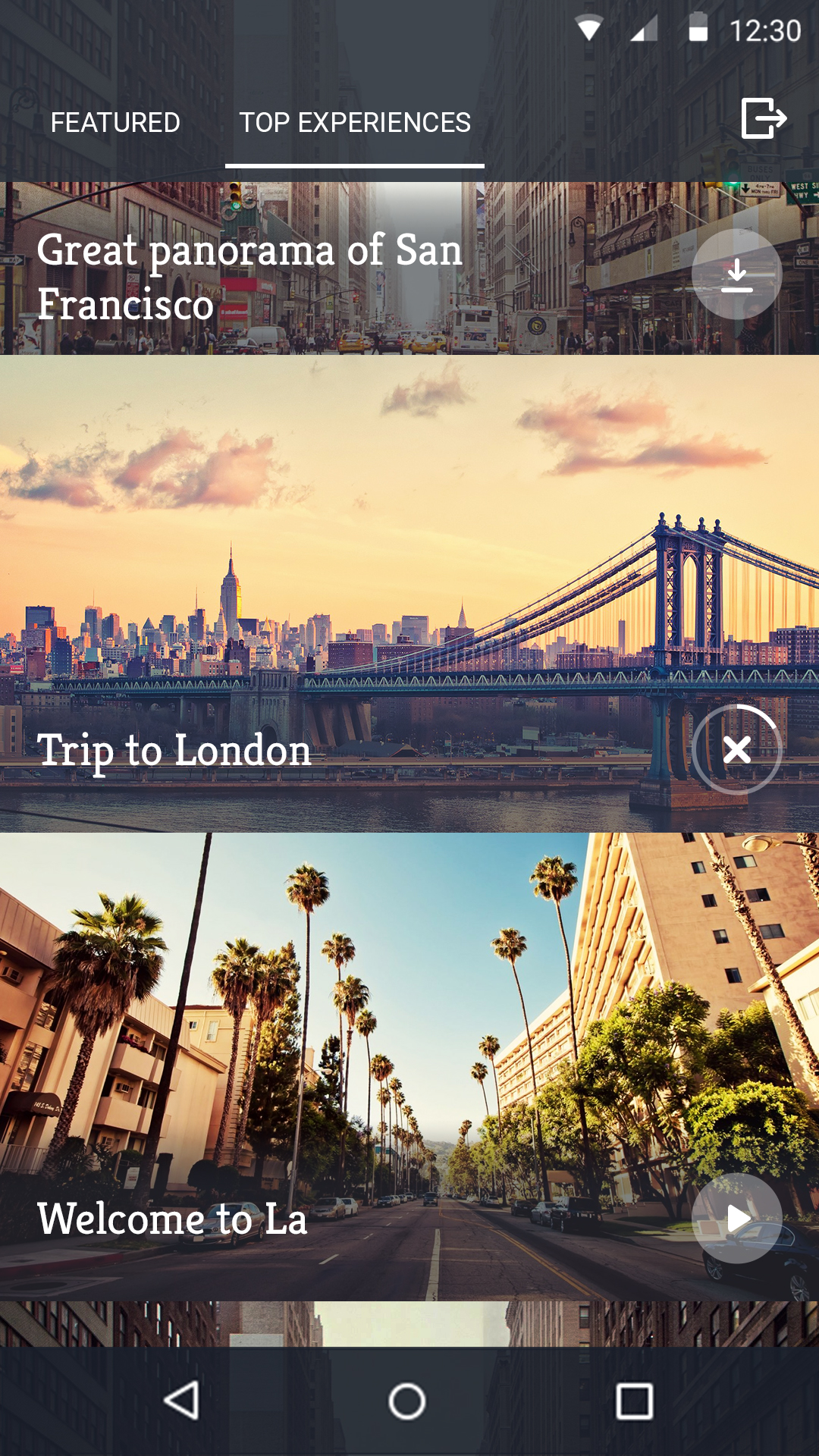This image displays a user interface of a trip planning application. The user interface contains gray bars at both the top and bottom of the screen. At the top of the interface, there are two tabs labeled "Featured" and "Top Experiences," accompanied by a logout icon towards the right. Below this, the screen prominently displays a section titled "Great Panorama of San Francisco" with an associated download button.

Further down, we see a section labeled "Trip to London," featuring an image likely depicting London Bridge. Next to this image, there are two icons: an 'X' for canceling the download and a circular progress bar indicating the ongoing download status.

At the bottom of the interface, there's a section named "Welcome to LA," which includes an image of a landscape in Los Angeles, showcasing trees and buildings, along with a play button to the right of the image. Each of these sections appears to showcase different destinations, providing visual aids and interactive options for the user.